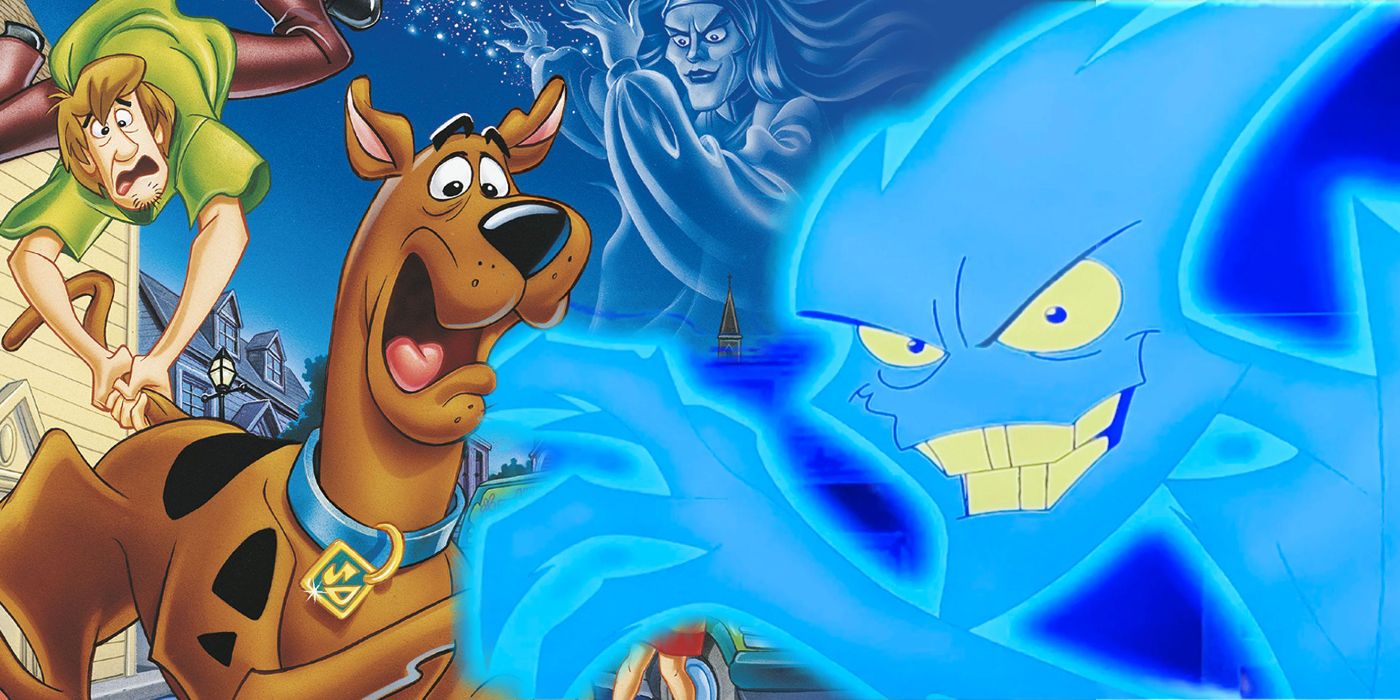The image is a vivid and dynamic scene from a Scooby-Doo cartoon. In the foreground, Scooby-Doo is prominently displayed on the left, wearing his familiar blue collar adorned with a gold tag. He has a frightened expression with his mouth wide open. Positioned closely behind him, Shaggy is grasping Scooby's tail as they appear to be in mid-flight, with Shaggy clad in his signature green shirt and brown pants. His anxious face adds to the sense of urgency and fear in the scene.

To the right of the image, there are two spectral figures that heighten the spooky atmosphere. One ghostly figure resembles a sorceress, her silhouette and shadow giving her an ominous presence in the sky. She appears ethereal with a mix of blue and white tones. Below her, a menacing blue monster with yellow eyes and a lightning bolt-shaped form grins deviously. This creature has sharp, jagged features, including lightning-like fingers and a lighter blue glow that amplifies his eerie appearance.

In the background, a couple of houses can be seen, grounding the scene in a typical Scooby-Doo setting where the supernatural meets everyday life. The sky serves as a backdrop, merging seamlessly with the sorceress figure, enhancing the surreal quality of the scene.